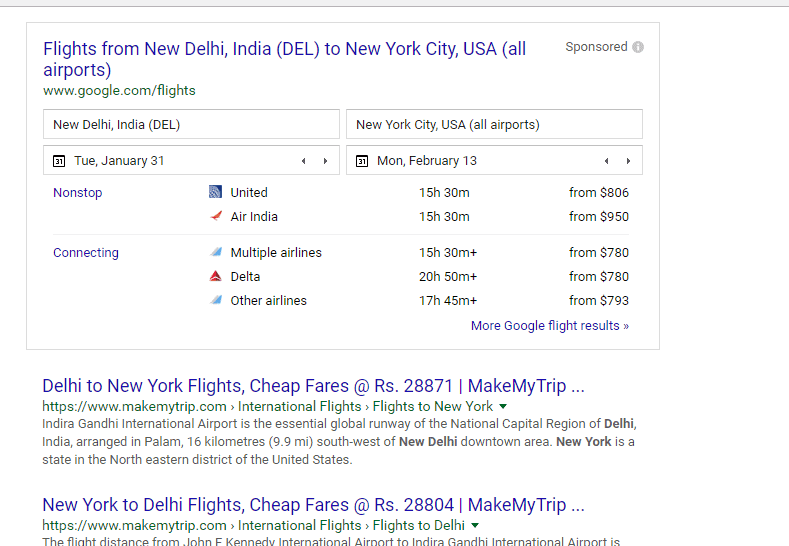Here is a detailed, cleaned-up caption for the provided image:

---

The image is a screenshot of a Google search page focusing on flight information. The top of the image includes a truncated grey bezel, with the same cut-off appearing on both the left and right sides. Dominating the top section within a thin grey-bordered rectangle is bold blue text detailing the search query: "flights from New Delhi, India (DEL) to New York City, USA (all airports)."

Below this, in blue font, the URL "www.google.com/flights" is displayed. The main section beneath the URL is divided into four distinct rectangles. The first rectangle on the far left indicates the departure location, "New Delhi, India (DEL)," while the adjacent rectangle to the right specifies the destination, "New York City, USA (all airports)." The second rectangle on the left features a calendar date marked with a bold black "31" and labeled in grey text as "Tuesday, January 31st," accompanied by left and right arrows for date adjustments. The rightmost rectangle mirrors this format but for the return date, indicating "Monday, February 13th" or "Mon-13-Feb" with left and right arrows for date scrolling.

Beneath these details, several flight options are listed. Non-stop flight options are highlighted first, with specific airlines and timings:

- United Airlines, marked by its symbol, offers a non-stop flight of 15 hours and 30 minutes starting at $806.
- Air India, symbolized by an orange swish, also presents a non-stop flight of 15 hours and 30 minutes with a starting fare of $950.

The section continues with connecting flights in blue text:

- Multiple airlines offer a connection flight of 15 hours and 30 minutes, starting from $760, indicated by a blue swish.
- Delta Airlines, represented by a red triangle, provides a connecting flight of 20 hours and 50 minutes from $780.
- Other airlines, marked again with a blue swish, have a connecting flight of 17 hours and 45 minutes starting at $793.

At the bottom right of this section, hyperlinked dark blue text reads "More Google flights results" followed by a double arrow pointing to the right.

Below these search results, two additional websites are listed in bold blue text:

1. "Delhi to New York flights cheap fares at RS.28871 | MakeMyTrip."
2. "New York to Delhi flights, cheap fares at RS.28804 | MakeMyTrip."

---